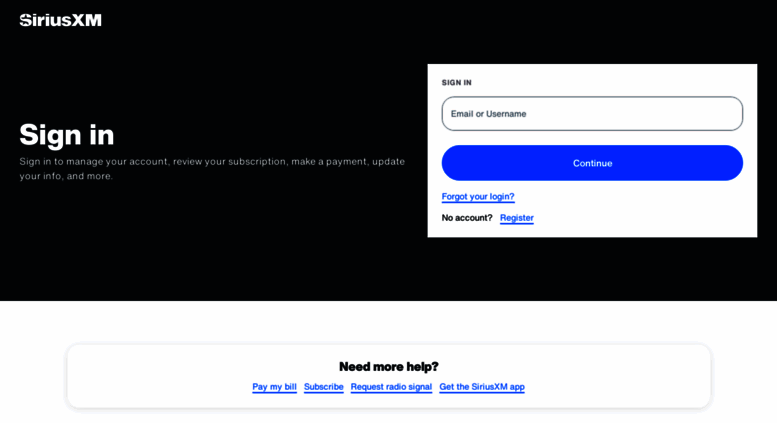This image is a screenshot from the Sirius XM website homepage. Dominating the background is a sleek black box, creating a striking contrast with the website elements. In the top left corner, the Sirius XM logo is prominently displayed in crisp white text, reading "Sirius XM."

Descending from the logo, the black space eventually transitions into an interface section featuring various text elements. The focal point of this section is the "Sign In" header followed by smaller text instructions stating, "Sign in to manage your account, review your subscription, make a payment, update your info and more." 

To the right of this header lies the sign-in form. It consists of a field labeled "Email or Username," and directly below, a blue button designed as a long, skinny rectangle with rounded edges, bearing the label "Continue."

Further down the interface are additional interactive text links in blue. There is a "Forgot your login?" link and a question prompt "No account?" followed by a "Register" button for new users. 

At the very bottom of the image, more blue text options are available, including "Pay My Bill," "Subscribe," "Refresh My Radio," and "Get the Sirius XM App," all designed to assist users with various needs.